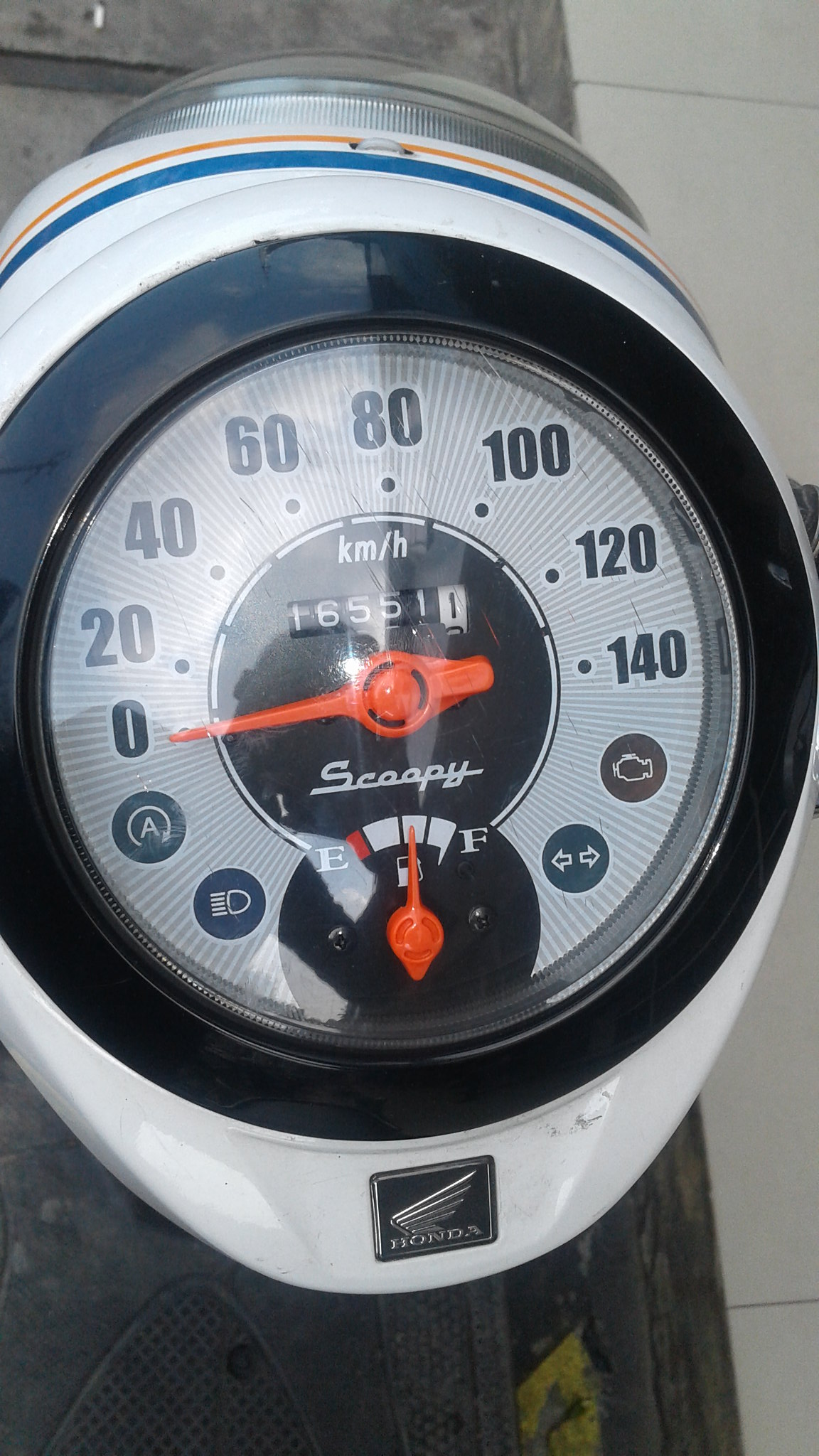The image features a detailed close-up of a speedometer and odometer, possibly belonging to a bicycle or another vehicle, as the specific context is unclear. The device is set against a background of white square tiles on the right and appears to be placed on a surface made of grayish leather or metal. 

The exterior casing of the speedometer is white plastic, giving it a very clean and pristine look. Prominently displayed on the bottom part of the gauge is a small black box with the Honda logo, including a silver bird's wing emblem.

The central part of the speedometer consists of a thick black circular border surrounding the actual gauge, which is protected by a glass cover. The speed scale ranges from 0 to 140 kilometers per hour, marked in increments of 20. An orange needle is currently pointing at 0.

Inside this main gauge, there is a smaller black circle at the center, with "kilometers per hour" written at the top in white text. Below this text, the odometer reads 600,551, indicating the distance traveled. At the very bottom of the gauge, a fuel gauge is visible, with the needle positioned halfway between empty and full.